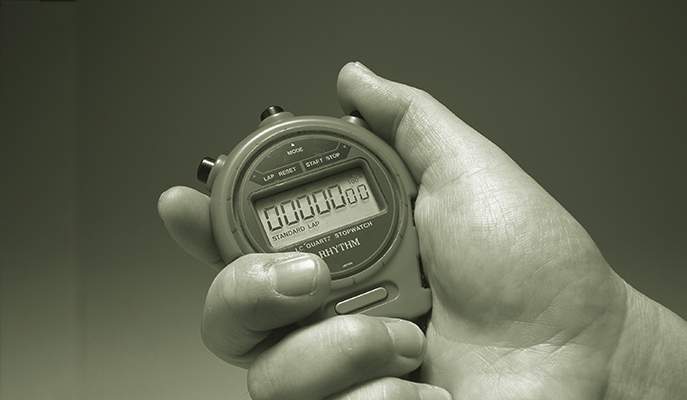The black-and-white photograph features a close-up of a man's hand, characterized by its slightly chubby appearance and short nails, emerging from the bottom right corner and holding a digital stopwatch near the center of the image. The hand appears to be of Caucasian skin tone. The stopwatch is plastic with a circular face and a rectangular digital screen displaying the digits "00:00:00.00." It has three black buttons on the top labeled "Mode," "Lap," "Reset," "Start," and "Stop," and additional text reading "quartz stopwatch" and "Rhythm." The background consists of varying shades of gray, transitioning from darker at the top to lighter at the bottom, creating a simple and uncluttered backdrop that emphasizes the solitary hand and stopwatch. This minimalistic and straightforward image could be suitable for use in an online clipart repository or on a sports-related website.